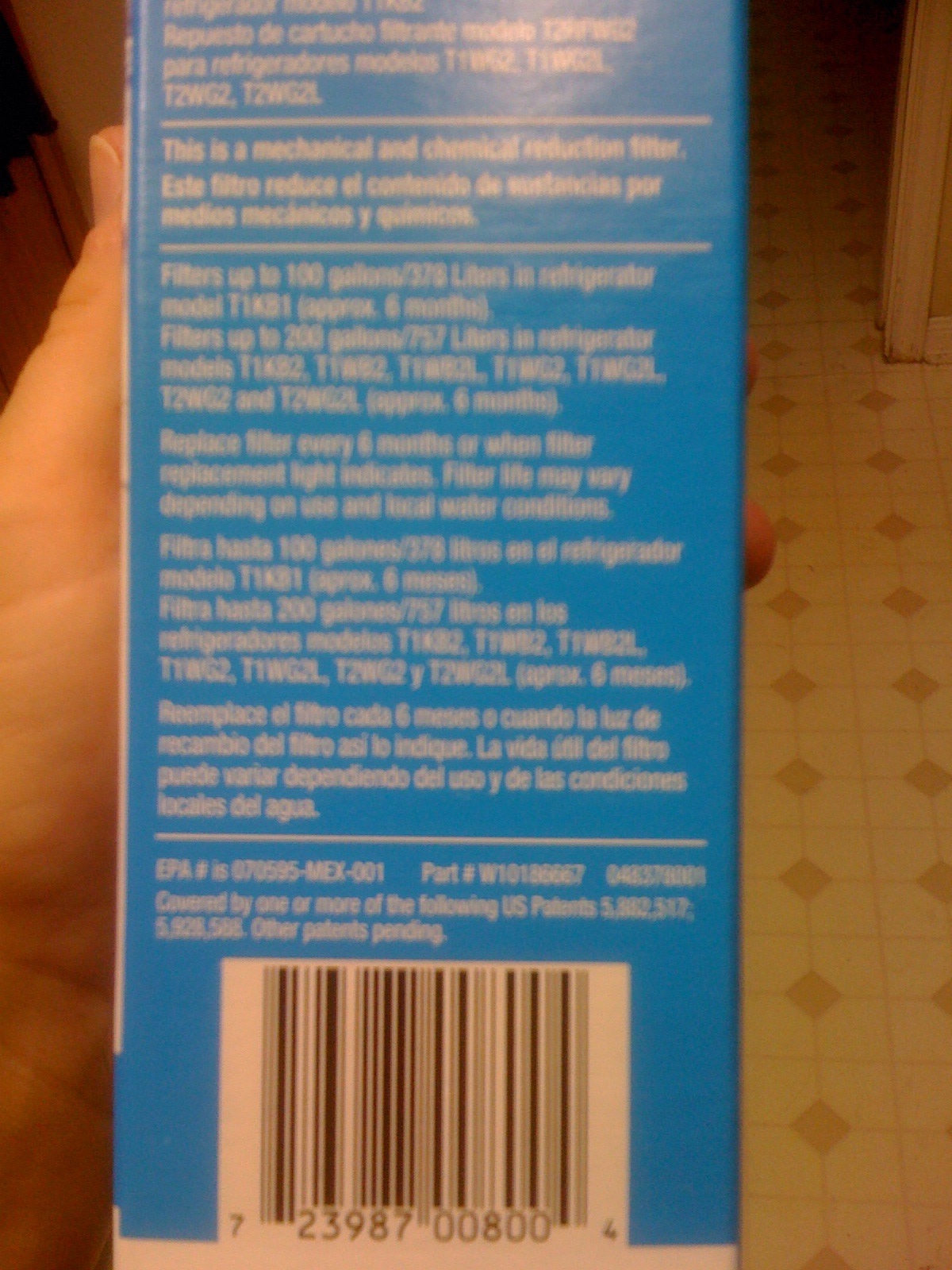The photograph portrays a close-up view of a blue cardboard box, held by a white hand with short nails, in a slightly blurred and out-of-focus image. The box is positioned in such a way that the narrow side with text is visible, albeit challenging to read due to the blur. At the top of the box, white text reads "This is a mechanical and chemical reduction filter," followed by detailed instructions and product information, including, "Filters up to 100 gallons, 378 liters in refrigerator model T1KB1 approximately six months. Replace filter every six months or when filter replacement light indicates. Filter life may vary depending on the use and liquid water conditions. Covered by one or more of the following U.S. patents 5882517, 5928566; other patents pending." The bottom of the box features a UPC code numbered 723987008004. The person holding the box is standing on a white linoleum floor adorned with brown or pink diamond patterns. The image also captures a hint of a door frame in the background.